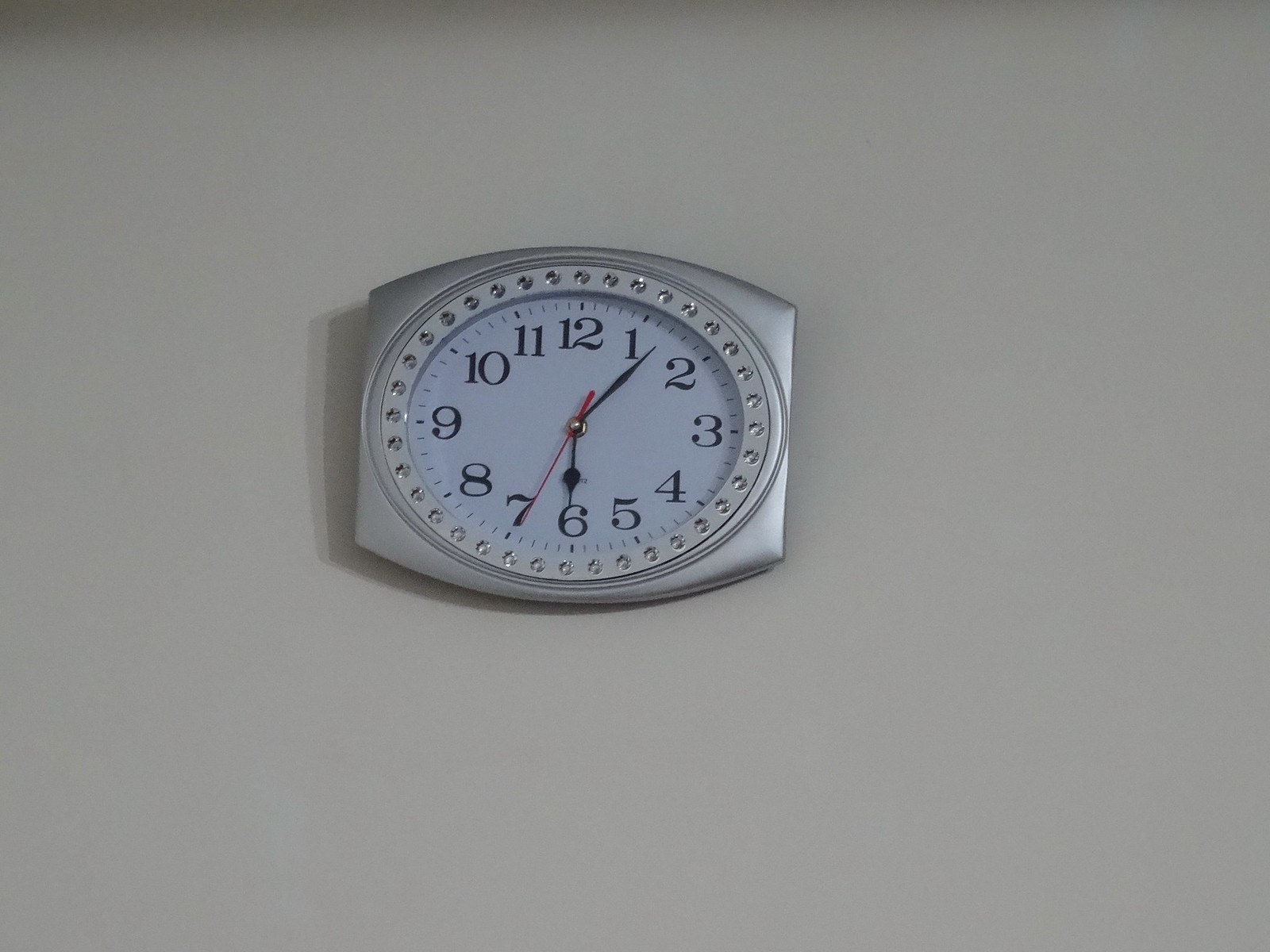The image showcases an elegant, silver-framed, analog clock mounted on a wall. The wall has a subtle beige hue, though lighting variations might give an impression of darkness at the top. The clock itself has an oval shape with squared ends, reminiscent of a football. Its silver rim is adorned with what appear to be small, glittering fake diamonds, adding a touch of sophistication. The clock face is white, featuring Roman numerals from 1 to 12 in a traditional fashion. The time indicated is approximately 6:07, marked by two black hands for the hour and minute, and a slender red second hand. The clock is encased in a slightly larger, polished silver exterior that enhances its overall sleek and modern appearance.